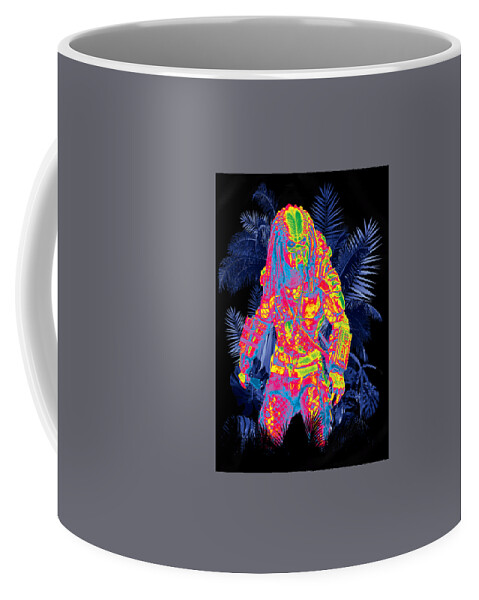The image depicts a 3D-rendered coffee mug with a white handle on the left side. The mug's exterior is a matte, medium-toned gray, while the interior is glossy white, matching the upper edge of the mug. Prominently featured on the gray exterior is a black rectangular section containing an image of the Predator from the Predator movies. The Predator is depicted in a thermal imaging style, showing tones of bright yellows, oranges, reds, greens, and blues, giving it a vivid, psychedelic feel. The background within the rectangle showcases large, dark blue palm branches and other plant elements, adding to the visual complexity. The overall aesthetic suggests a low-quality or homemade sticker, reminiscent of bootleg merchandise, yet it effectively captures the iconic heat-vision imagery from the film.